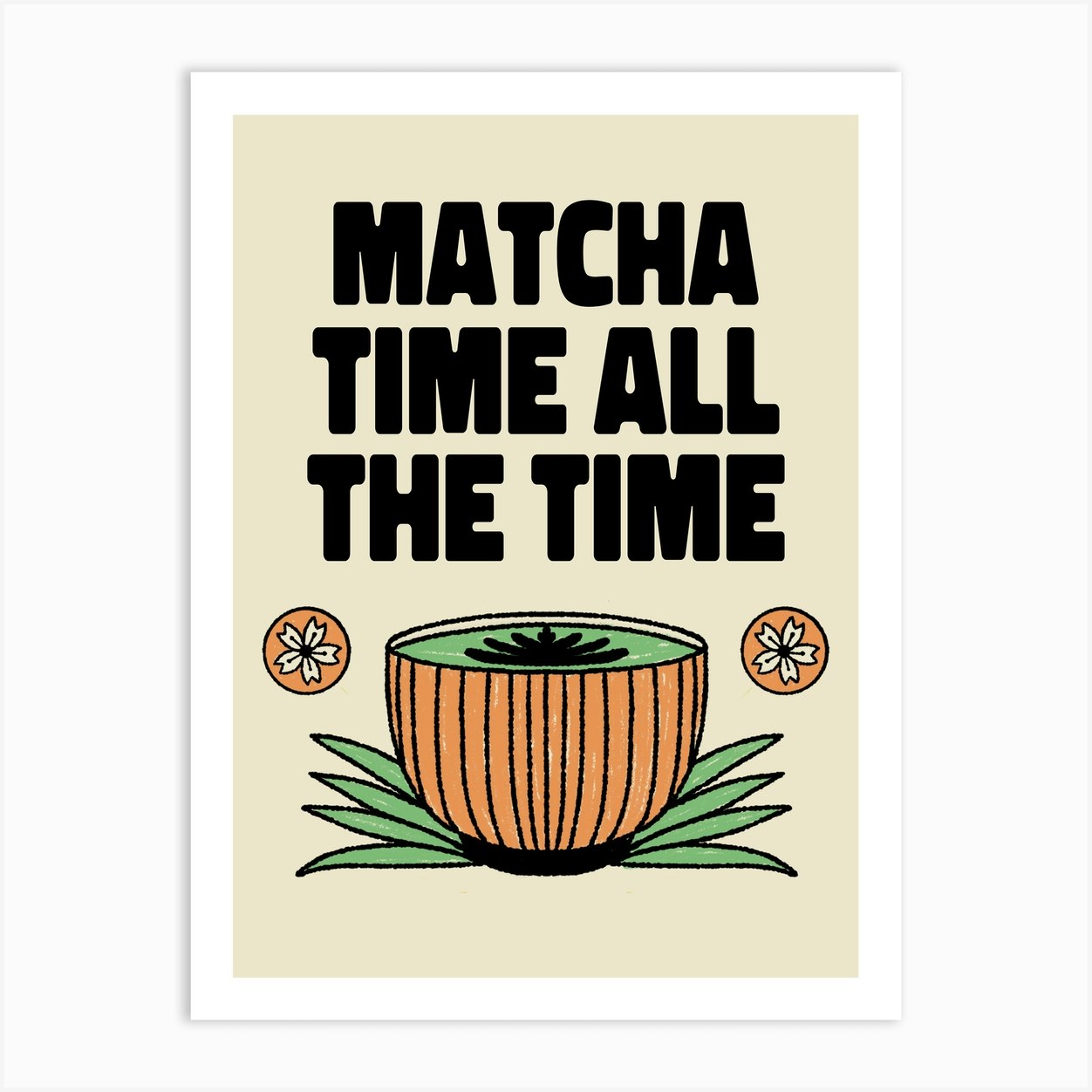The advertisement features a beige background with prominent black text at the top that reads, "Matcha Time All the Time". Below the slogan is an intricately designed, hand-drawn image of a cup filled with green tea. The cup, striped in shades of brown and orange with a black base, sits atop a layer of green leaves. On either side of the cup are circular orange discs featuring detailed leaf designs. The green tea inside the cup displays a black leaf pattern, as if artfully crafted by a barista. The overall presentation has a warm, inviting feel, evoking a sense of artisanal quality and attention to detail.